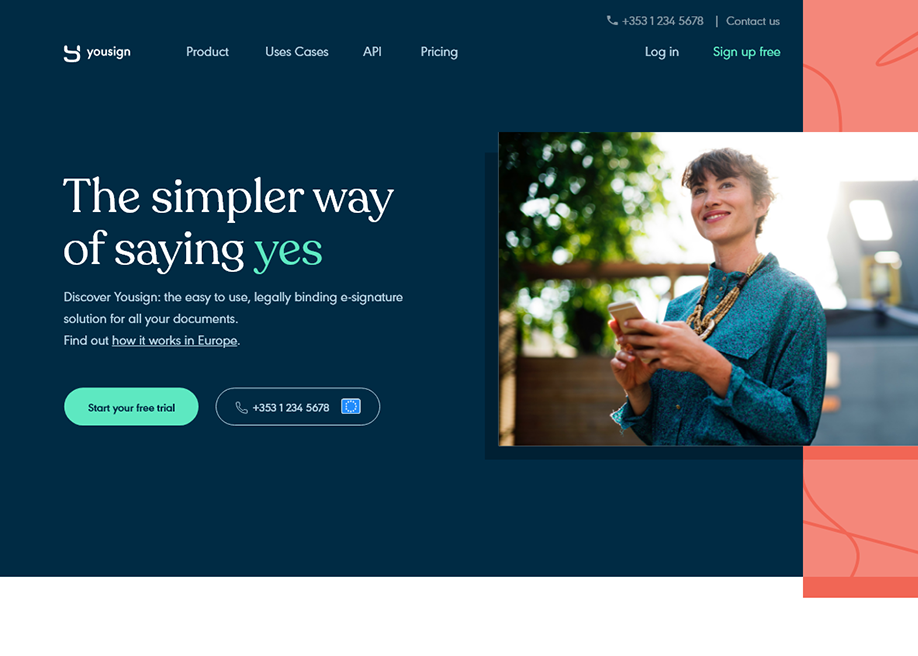The image is a horizontal webpage layout for a product or service, designed with a distinctly divided background. The left two-thirds feature a dark blue backdrop, while the right side transitions into a light red that almost appears orange, enhanced with subtle lines. Prominently displayed on the right is a smiling woman with short brown hair. She is dressed in a stylish blue and black patterned button-down shirt and accessorized with necklaces, holding a smartphone in her hand. The text on the webpage prominently reads, "The simpler way of saying yes," with "yes" highlighted in green. Beneath that, in smaller white text, it says, "Discover USIGN, the easy to use, legally binding e-signature solution for all your documents. Find out how it works in Europe." This webpage promotes an e-signature service called USIGN, emphasizing its user-friendly and legally compliant features.